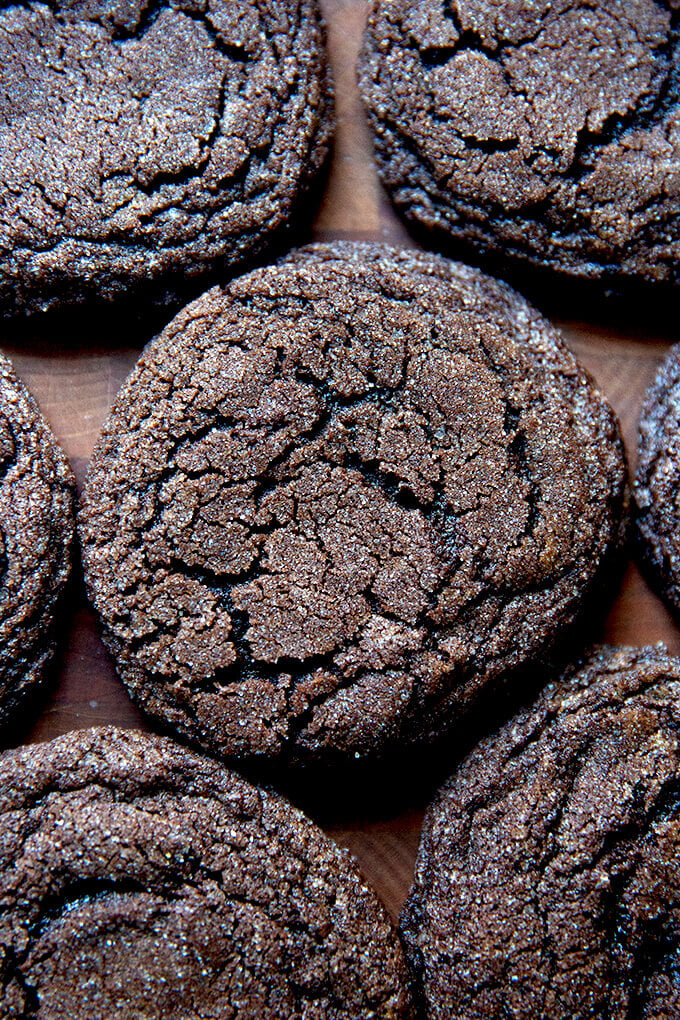This close-up image highlights a cluster of rich, dark chocolate cookies resting on a wooden surface. The cookies have a dense, chewy texture, resembling brownies due to their deep brown, almost black coloration on the sides. In the center of the picture, a single cookie is shown in its entirety, complete with visible cracks and a sprinkling of white sugar crystals. Surrounding this central cookie, fragments of six additional cookies are positioned closely, with two above, one to each side, and two below, all partially cut off by the camera's frame. The wooden surface beneath the cookies features visible grooves, adding a rustic touch to the composition. This detailed arrangement and the visual appeal of the cracked, sugar-dusted tops suggest these cookies are both rich in flavor and tempting to the taste.